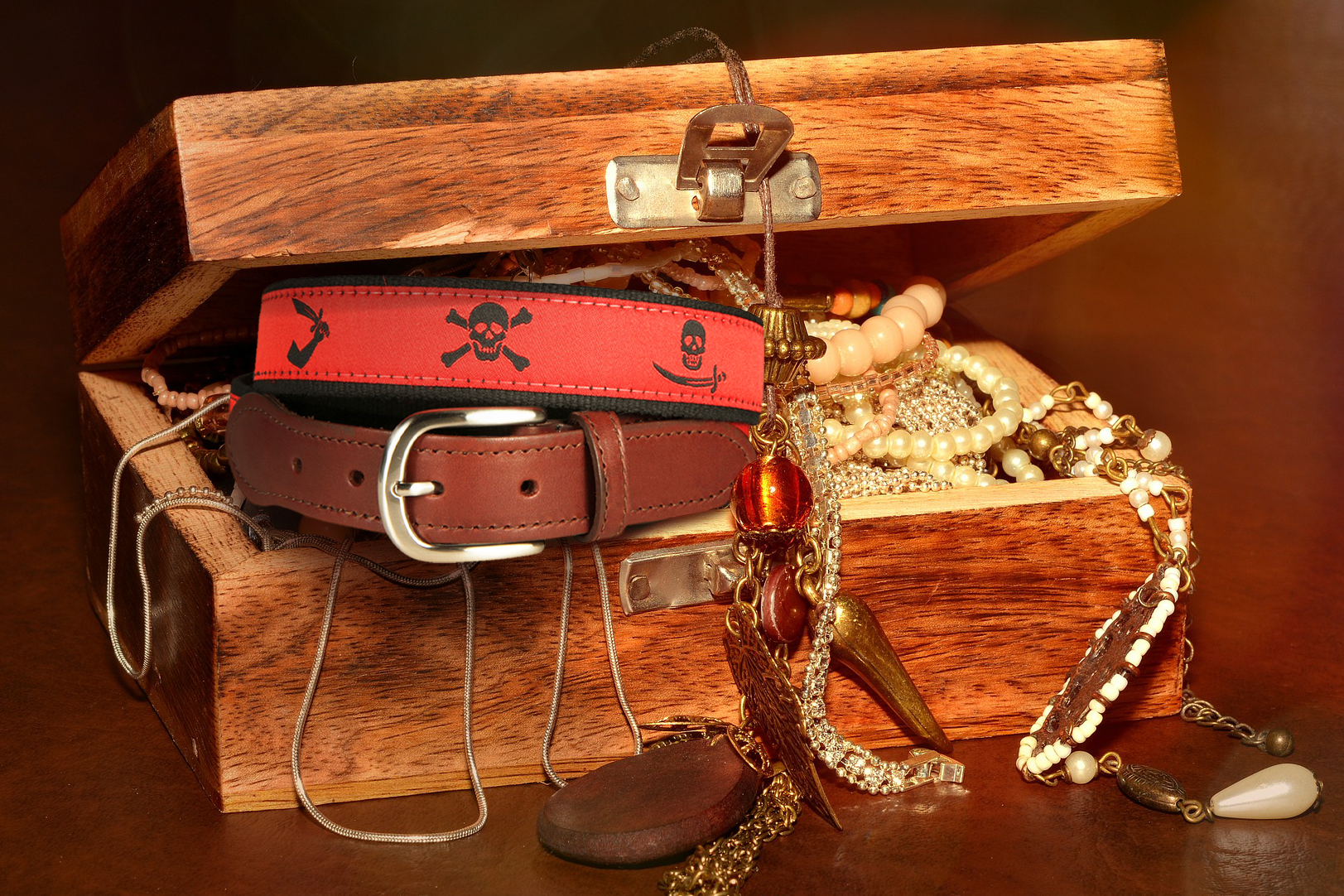This image features a small, wooden jewelry box, styled to resemble a pirate's treasure chest. The box is a natural shade of wood, neither too dark nor too light, and boasts a brass clasp that appears unable to close due to the box being overfilled. The chest sits on a brown surface with no discernible background. Inside, the box holds an assortment of jewelry and two belts. One belt is plain brown with a silver buckle, while the other is red with black skull and crossbones prints, detailed with a diagonal sword and an arm holding another sword. Jewelry is spilling out of the box, including gold necklaces with white and orange beads, and large, off-white pearls overlaying a smaller string of pearls. Some pieces are inside the chest, while others dangle from it, adding to the sense of overflowing treasure.